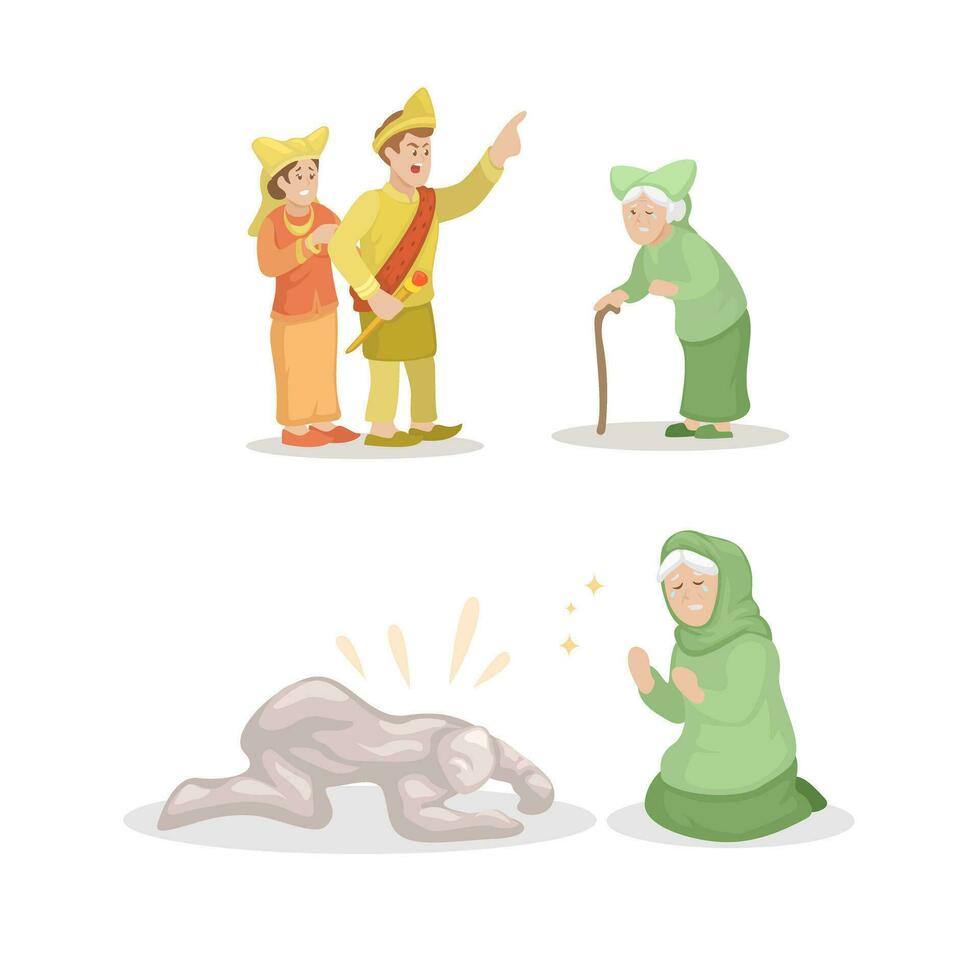This is a set of two vibrant color illustrations, arranged vertically, showcasing dramatic scenes involving the same central figure: an old woman with white hair in a green outfit. The artwork features a distinctly preschool cartoon style.

In the top illustration, the old woman is leaning on a brown cane and appears to be tearful, confronting a couple. The man, positioned on the right, has blonde hair and is depicted with an authoritative, angry expression. He lifts his left hand as if remonstrating and holds a scepter in his right. He is adorned in a crown or headdress, a gold shirt, green kurta, pants, and gold slippers, with a red sash completing his regal attire. Standing beside him, a young woman in fancy clothes and a gold headdress has an unreadable expression, possibly of concern or distress. She wears an orange shirt, gold necklace, and shoes.

The scene below captures the old woman kneeling and weeping in front of a mysterious figure that seems to be either a golem or a ghost, with lines around it indicating an emanation of power. This figure, which could be stone or wax, remains ambiguous due to the illustrative style. The emotional contrast between the authoritative confrontation above and the old woman's sorrowful submission below is stark and evocative.